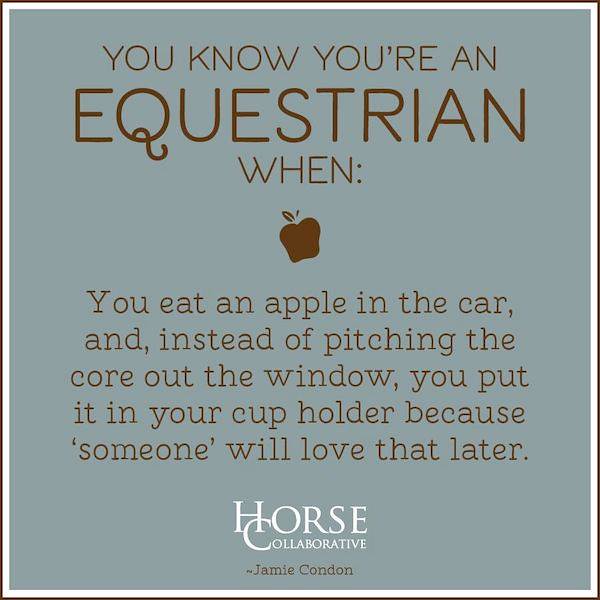The image predominantly features text framed by a thin black pinstripe outer border and a slightly wider white inner border, set against a slate gray background. Centered at the top, it reads "You know you're an equestrian when..." in large, deep brown text. Below this header is a stylized illustration of a brown apple. The main body text, also in deep brown, continues: "You eat an apple in the car, and instead of pitching the core out the window, you put it in your cup holder because someone will love that later." At the bottom, in white text, is the attribution "Horse Collaborative, Jamie Condon," with the 'H' of "Horse" and the 'C' of "Collaborative" slightly overlapped. The overall style suggests a motivational or humorous poster, suitable for sharing on social media platforms like Pinterest or Facebook. The design is clean and the text is well-spaced, ensuring legibility. The color palette mainly includes shades of brown, white, and slate gray.